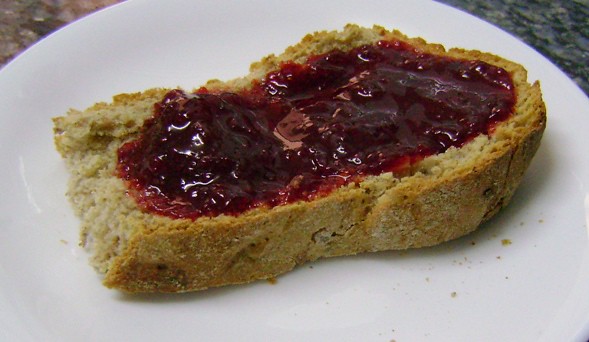This close-up photograph features a half piece of crusty, light tan to brown bread, generously spread with a thick, shiny, dark red jelly, possibly strawberry or raspberry. The bread, dusted with a bit of white flour, is centered on a plain white porcelain plate that takes up most of the image, curving into the top left and right corners. Both the bread and plate sit on a marble countertop, characterized by various red, pink, white, and green flakes. Despite the dark lighting of the image, detailed textures and elements like the possible fruit pieces in the jelly and the face-like reflection in the spread are distinctly visible.